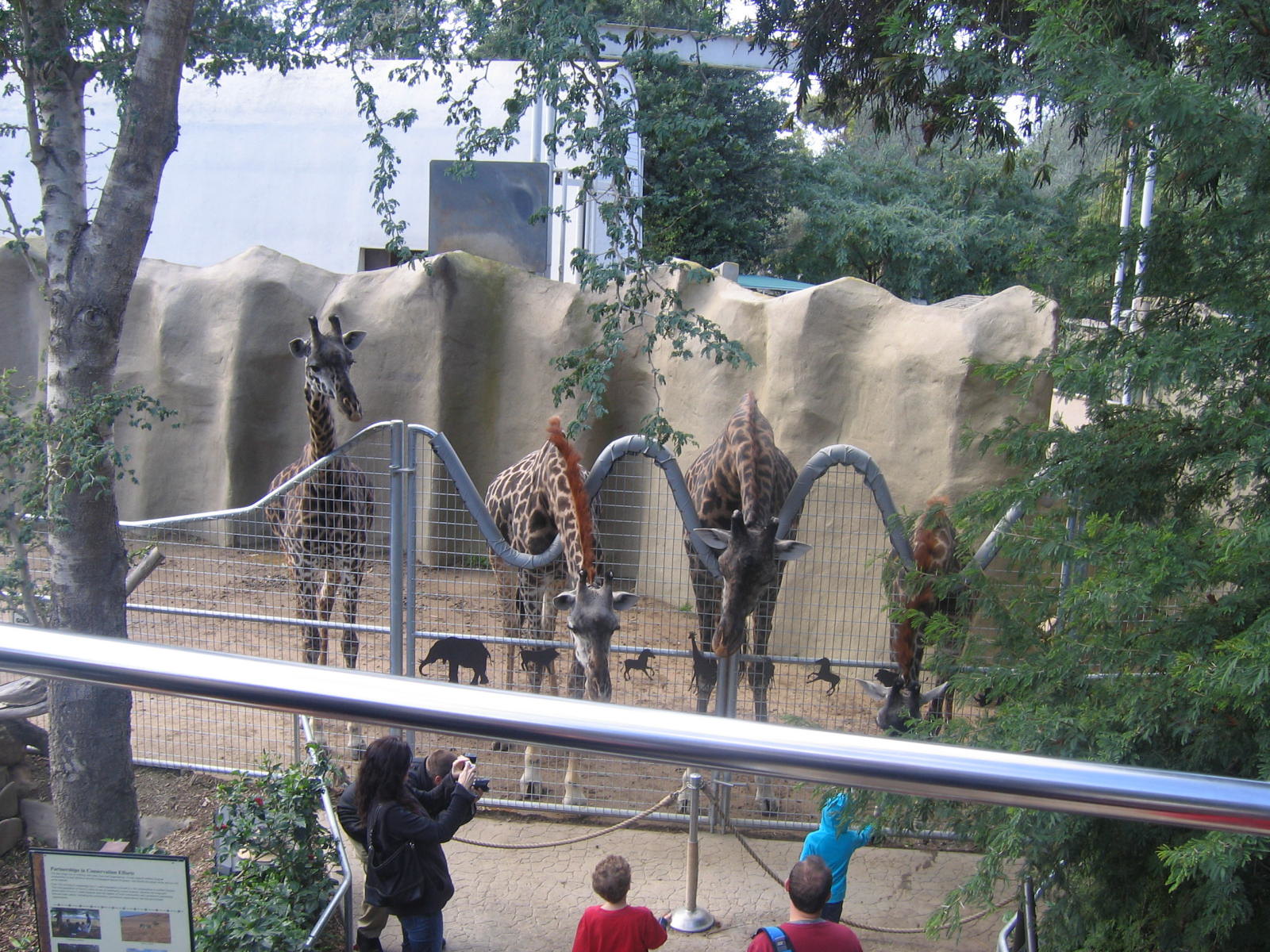The image showcases a bustling zoo scene viewed from an elevated perspective, with a metal railing in the foreground. Below, a small enclosure houses four majestic giraffes against a backdrop of an artificial rock wall. A metal fence with a distinctive undulating design allows the giraffes to lean over into the viewing area where numerous families, including a woman with a camera and several children, eagerly observe and photograph the animals. One giraffe is particularly engaging, craning its neck over the fence, seemingly seeking interaction or food. The enclosure is flanked by lush trees and bushes, adding a touch of natural greenery. To the left, a sign provides information about the giraffes, and a white building is visible in the background, completing this lively and detailed zoo snapshot.